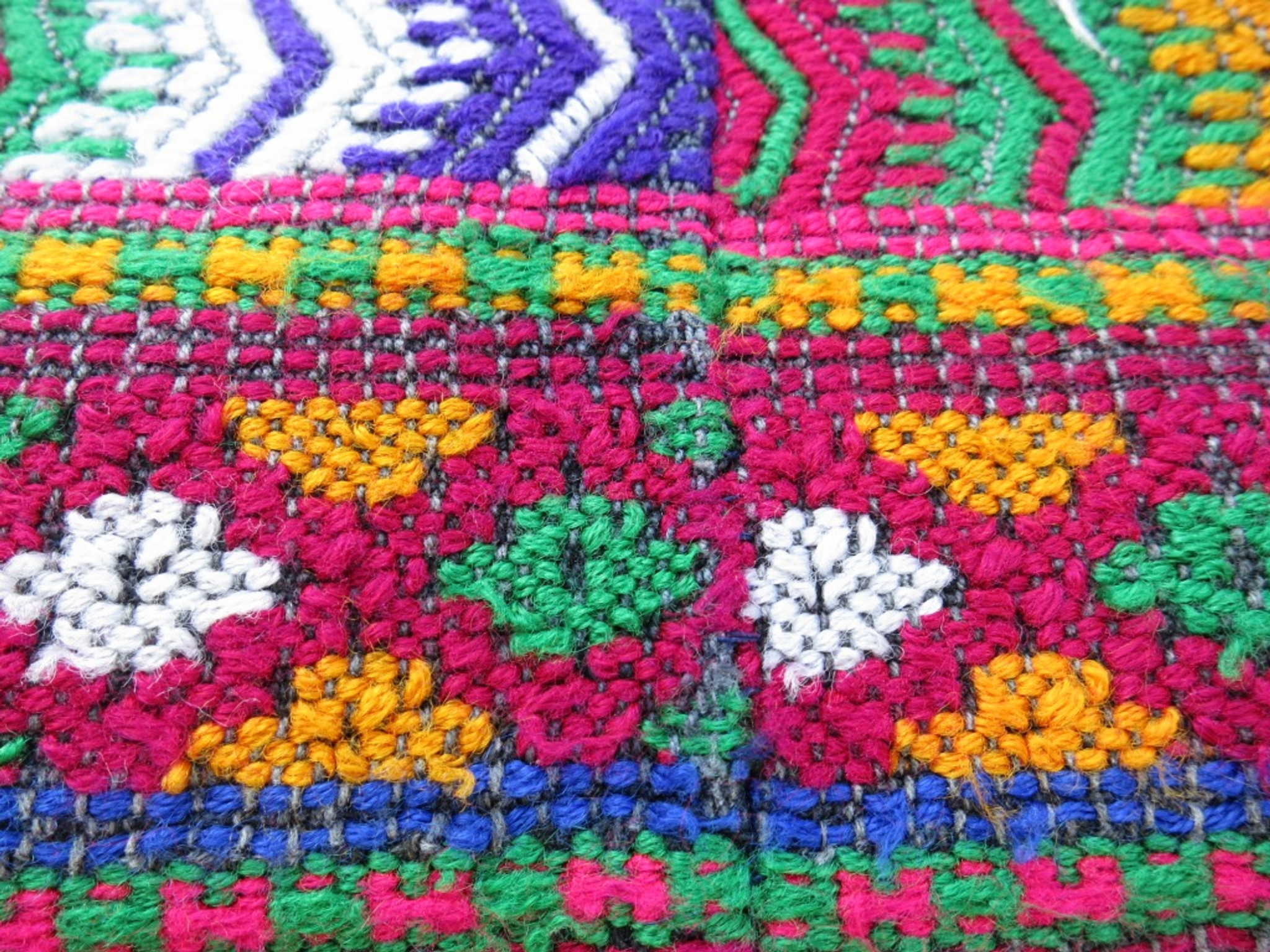This is a detailed close-up photograph of a meticulously handcrafted crochet piece, characterized by an intricate pattern of vibrant colors and designs. The artwork features two prominent banners, one positioned centrally and one at the bottom border, both incorporating rows of purple threads. The upper section of the piece showcases lines of hot pink threads, interspersed with chevron-style patterns in greens, whites, purples, pinks, and yellows, creating a striking visual effect. Between the two banners, there's a row of pink flowers with alternating white and green centers, adding a touch of floral elegance. Additionally, various sections of the crochet highlight horizontal stripes and bands, including a green band adorned with pink letter H's, a royal blue band, and a wide pink band rich with green, gold, and white shapes. The detailed embroidered designs and the seam running down the middle further accentuate the complexity and craftsmanship of this vibrant textile piece.